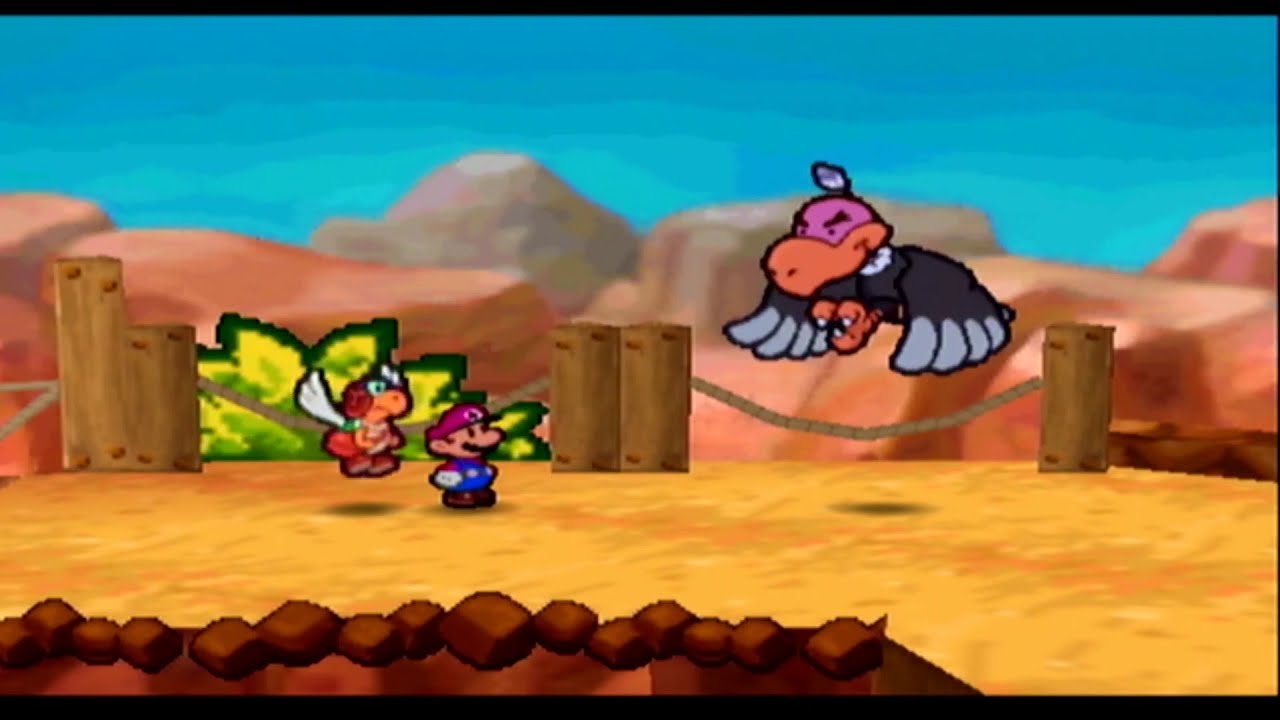In this detailed screenshot of a Super Mario Brothers video game, Mario, dressed in a blue jumpsuit with a hat that appears pinkish, stands on a sandy ground. The setting includes a foreground with rocks, while the backdrop reveals a range of brown and gray mountains beneath a vivid blue sky. Interspersed with these elements are wooden poles connected by ropes, forming a barrier that suggests a boundary or path.

To Mario’s left, a flying turtle-like creature with a black aviator cap and white wings hovers in the air. On the right looms a menacing giant bird resembling a vulture, characterized by its black body, gray-tipped wings, orange talons, an orange beak, and a pinkish head adorned with a solitary white feather. The bird's aggressive stance, with its talons extended forward, hints at an impending attack. Mario, facing toward the right, seems poised for the challenge, adding a dynamic tension to the scene.